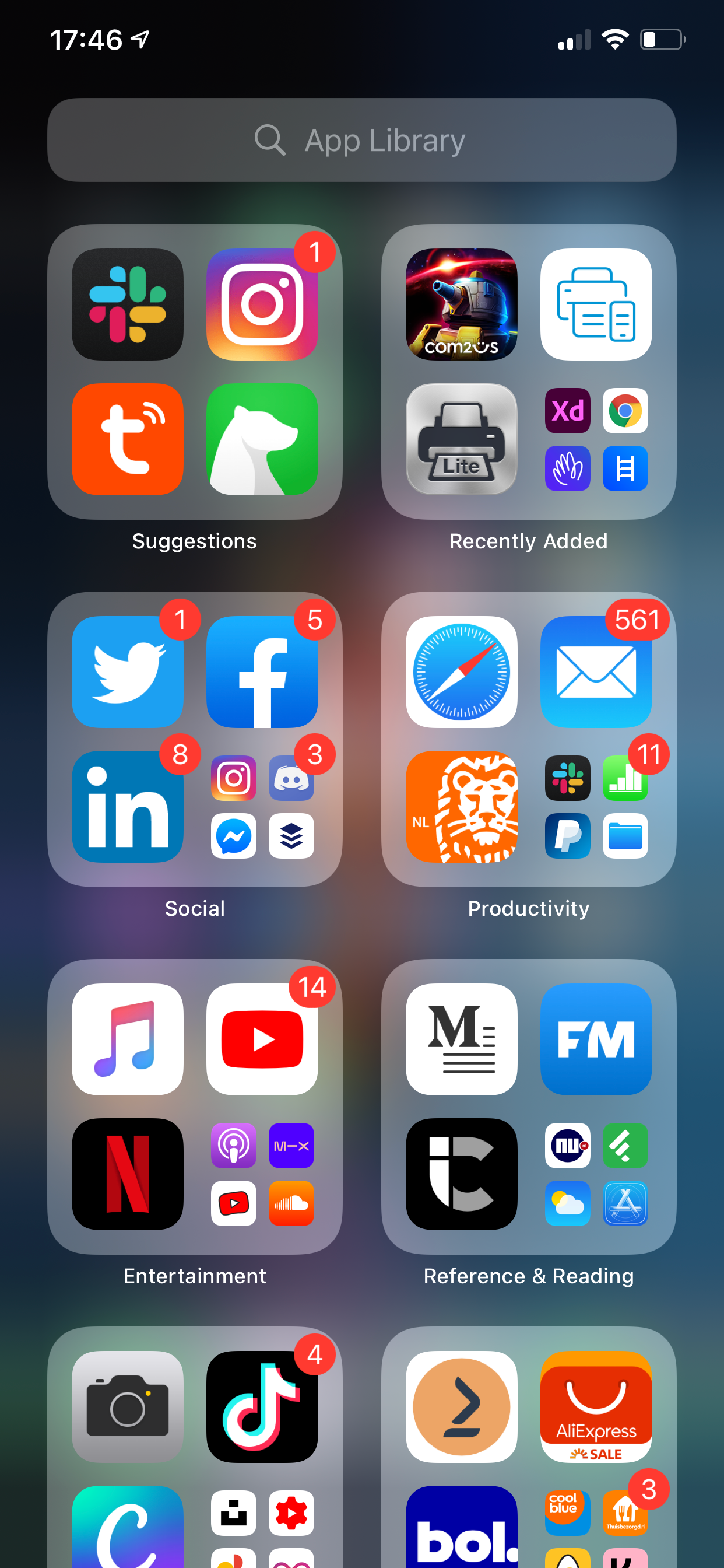This screenshot displays the screen of a person's smartphone with various app libraries and folders organized neatly. At the top left corner, the time is 17:46. On the top right, there are icons indicating cellular coverage bars, Wi-Fi connectivity, and battery status. The upper area of the screen features a gray rectangular search bar with a white magnifying glass icon inside it, labeled "App Library."

Below the search bar, several folders are visible:

1. **Suggestions:** This folder includes icons for Instagram, Tumblr, a green icon with a white polar bear outline, and another icon featuring blue, green, red, and yellow oblong shapes.

2. **Recently Added:** This folder contains icons for:
   - COM2 smiley face S
   - A printer icon
   - A printer icon labeled "Light"
   - XD
   - Google
   - A blue square with a white ladder
   - A dark blue square with a scribbled pattern

3. **Social:** This folder comprises icons for:
   - Twitter
   - Facebook
   - LinkedIn
   - Instagram
   - Discord

4. **Productivity:** This folder's icons include:
   - Safari
   - Email
   - An orange icon with a white lion and the letters "NL"
   - PayPal
   - A folder icon

5. **Entertainment:** The icons in this folder are:
   - Music
   - YouTube
   - Netflix

6. **Reference & Reading:** This folder features various icons including:
   - Weather
   - App Store
   - FM

Additionally, there are two folders at the bottom of the screen that are partially cut off, making it difficult to identify their contents.